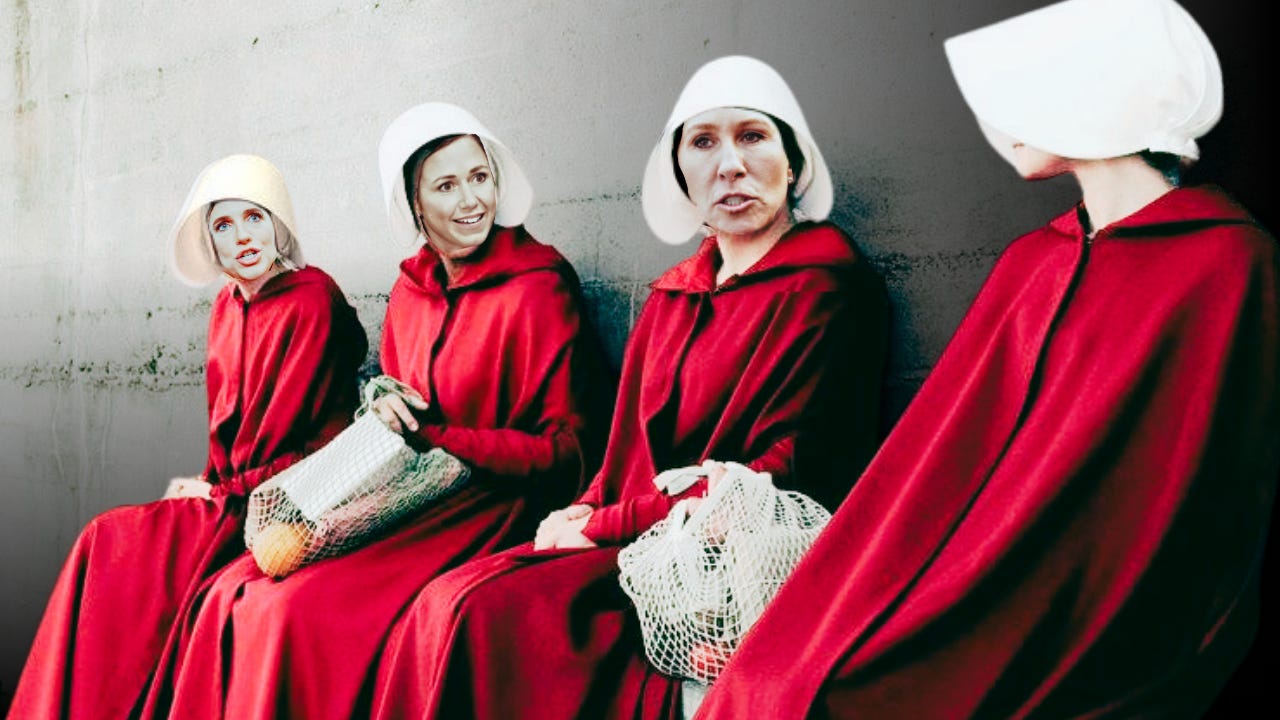The photo depicts a striking scene against a concrete wall featuring four women adorned in the iconic red robes and white bonnets of 'The Handmaid's Tale.' Their attire completely covers their bodies, making a stark contrast to the sparse background. Three of the women face the camera, their faces visibly edited, suggesting they could be well-known figures such as Marjorie Taylor Greene and Carrie Lake, while the face of the fourth woman is turned away, hidden from view. The women hold mesh bags containing various items, including what seems to be oranges and papers. This image, possibly a meme without any accompanying text, appears to satirize the extreme conservatism associated with Republican women, evoking the dystopian themes of the Hulu series. The surreal ambiance created by the red robes against the concrete backdrop further accentuates the jarring and possibly protest-laden narrative of the photograph.